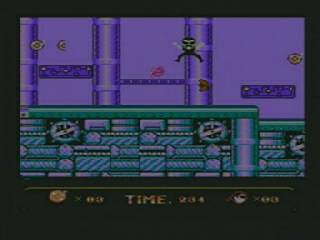The screenshot from the video game features a predominantly violet background with three prominent cylindrical pillars stretching vertically. Purple pipes intertwine horizontally between these pillars, adding to the complexity of the architecture. The pillars themselves are adorned with floating gold coin-like objects, either circular or half-circular, contributing to the game's rewarding elements. 

In the foreground, a character with distinct black features—black hair, eyes, mustache, shirt, pants, and shoes—strikingly contrasts with his gray and white skin. The character, who is notably smiling with a white dot on his mouth, is captured mid-jump, arms stretched out wide, projecting an air of triumphant effort. 

Beneath him is a green platform, shading into darker hues, embedded with teal and light blue gear-like objects and bricks. At the bottom of the screen, a legend reads "TIME 231," next to a close-up of a face and an icon denoting lives with “X00." The overall scene is vibrant and bustling with details, capturing the essence of arcade-style video gaming.